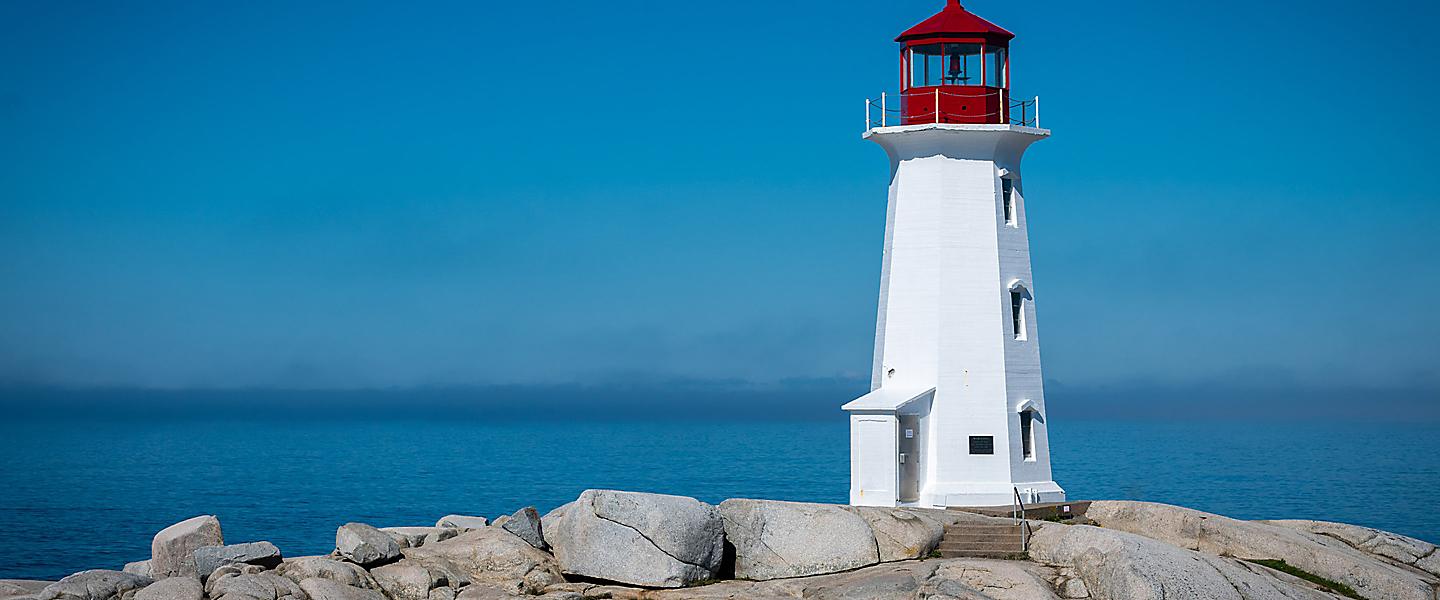This serene image captures a picturesque lighthouse perched on a segmented bed of gray and tan rocks at the edge of a vast body of water, possibly an ocean. The lighthouse, standing approximately four stories tall, features a stark white base and a striking red hexagonal cupola at its peak, which resembles a gazebo with white poles and chains encircling it. The calm, blue water stretches to the horizon, blending into a clear blue sky that gradually deepens in color. The lighthouse has three visible windows and a small door leading into the structure, accentuated by a small flight of stone steps and a railing that ascend a boulder beside it. The overall scene is wide-angle, capturing the tranquility of the setting with light grayish clouds forming near the horizon.